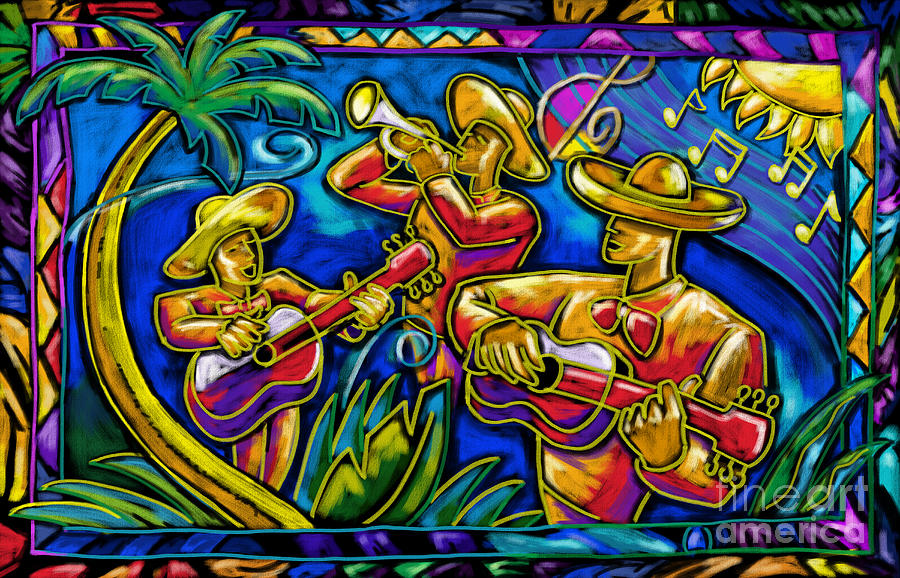The image is a vibrant and colorful rectangular mural depicting three Mexican musicians, arranged from left to right. The characters are painted in an artistic, non-realistic style with golden hues, giving them a distinct, almost bronze appearance. The person on the right is wearing a sombrero that obscures his eyes, a red bow tie, and is holding a downward-facing guitar with a pink neck and a body that is mostly purple with some pink, all outlined in light green. The middle musician is playing a trumpet aimed upward to the left. He wears a hat with the brim curving upward and holds the mostly white trumpet, which has a yellow hole with a black ring around it, with both hands, his elbows pointing outward. The person on the left, facing right, is holding a large guitar that features a white upper body and a purple and red lower section, the bottom fully purple. This musician also sports a brimmed hat curving upward.

In the background, a palm tree begins near the feet of the leftmost figure, curving towards the left and adorned with green leaves. The upper right corner showcases a bright yellow and orange sun, beneath which musical notes, in yellow, float. The entire backdrop is a gradient of blue and teal with swirling lines on the right side. At the bottom, vibrant plants grow in shades of yellow, green, and light blue. The image is signed with ghosted lettering in the bottom right corner, spelling "F-I-N-E-A-R-T," and underneath, in purple and pink, "America."